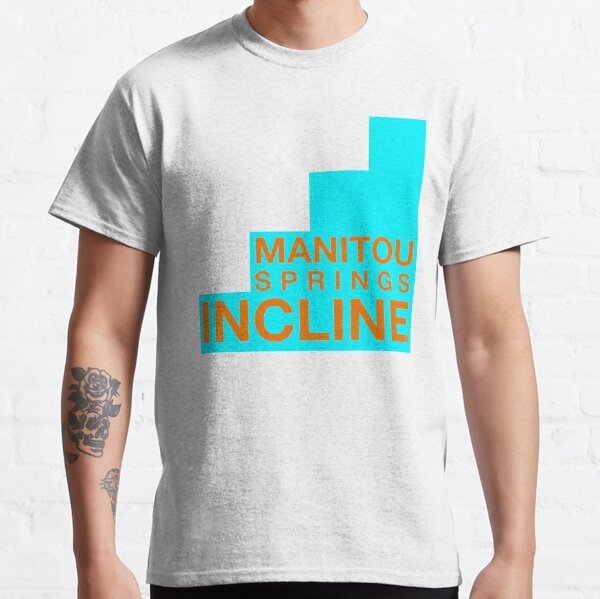In this outdoor photographic image, a man, who appears to be Caucasian with visible neck and arms, stands against a white painted brick wall. He is wearing a grey round collar t-shirt that extends just over his crotch. The t-shirt features an orange and blue graphic resembling a set of steps, with the text "Manitou Springs Incline" across three lines. "INCLINE" is in the largest font, while "MANITOU SPRINGS" is in a smaller font, all in capital letters. The man's right arm reveals a detailed tattoo of a rose over a skull, with the skull oriented left to right. Another tattoo, potentially of a cougar or wild cat, is partially visible on his inner forearm but not fully discernible. The lighting suggests the light source is coming from the left, casting soft shadows on the right side of the man's shirt and neck.